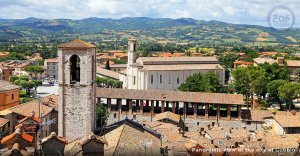This high-angle photograph captures a richly detailed panorama of a small urban area surrounded by natural elements. The image, presented in a small horizontal rectangle, prominently features a collection of human-made buildings with diverse architectural details. Most of the buildings have brown, triangular roofs, with walls painted in varying shades of white and cream. 

Central to the image, slightly left of center, is a stone tower with a small, roundish brown top and a pointed roof. The tower includes a significant archway window near the top. A roof extends rightward from the tower, under which appears to be a bridge connecting to the tower. In this same region, tiny figures can be seen walking around a gray area, indicating human activity. 

In the bottom right of the photo, additional brown roofs and some indistinct structures are visible. Above the bridge and towards the middle distance, a prominent white building with a steeple-like feature can be seen, possibly suggesting a church or significant public building, flanked by more trees and rooftops.

Beyond the urban cluster, the ground transitions into an verdant area with numerous green trees. This section leads further into the landscape where small hills rise, stretching across the entire background of the image. The scene is capped with a sky filled with clouds, adding depth and framing to this picturesque setting.